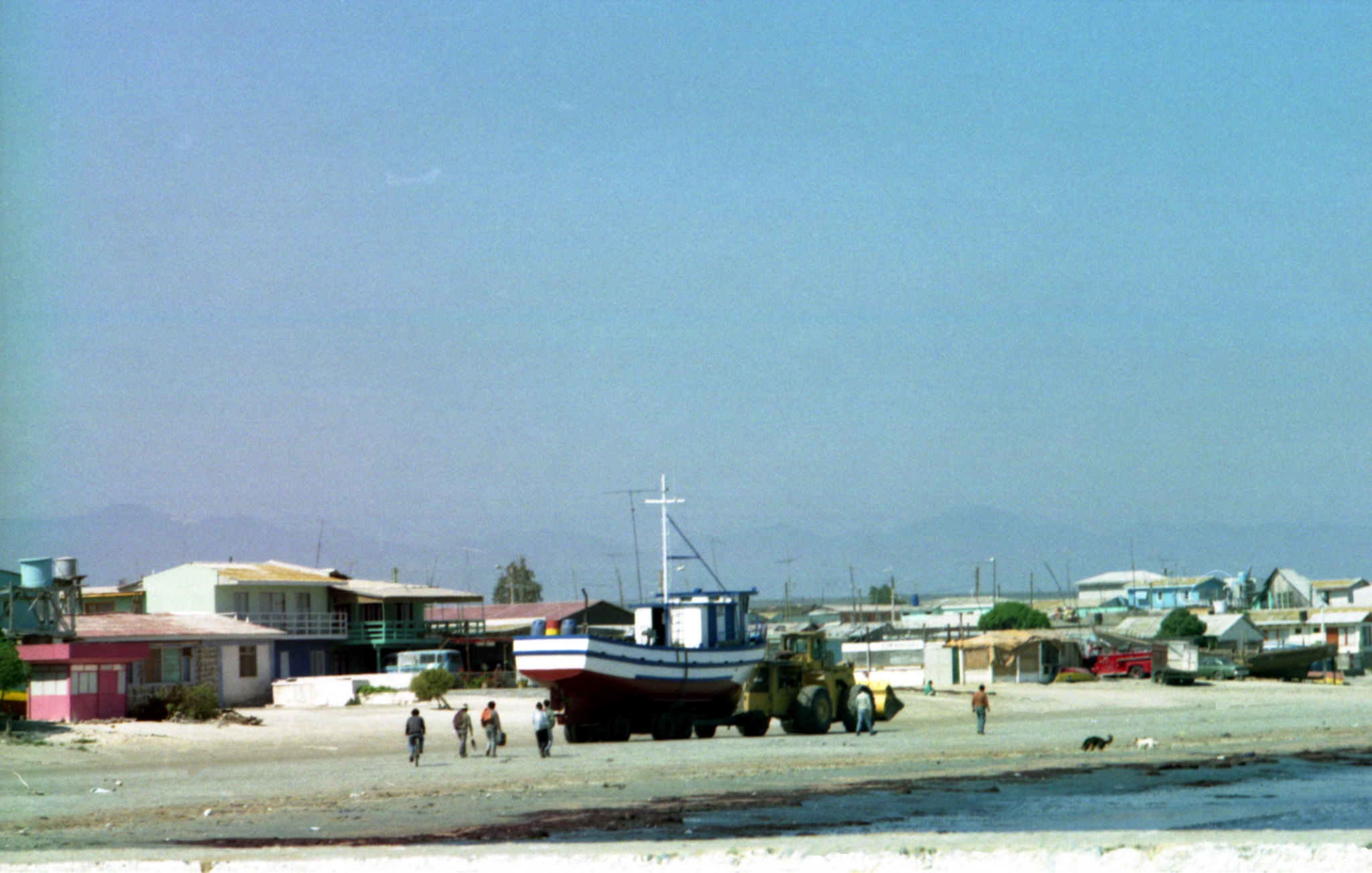In this outdoor beach scene, an overcast and slightly foggy sky stretches above a bustling shoreline. The distant hazy outlines of mountains frame the background, adding an element of grandeur to the view. A handful of houses in worn shades of blue, pink, white, and tan dot the landscape, their weathered facades telling stories of resilience.

At the center of the composition is a visually striking boat, mostly white with a red bottom and a blue stripe circling it. The boat, adorned with a large cross and a mast suggestive of a sail setup, is perched atop a tractor, being transported along the sandy shore. Some details hint at it being a medium-sized vessel, though opinions differ on its exact size. Surrounding this focal point, at least seven people are walking purposefully towards the boat, adding a sense of motion and anticipation to the scene.

In the foreground to the bottom right, a small patch of water glistens subtly. Nearby, a red pickup truck stands out against the sparse activity. A few cats roam freely near the shore, echoing the calm yet lively ambiance, while the muted colors of the sky and landscape blend harmoniously, capturing the serene beauty of this coastal tableau.